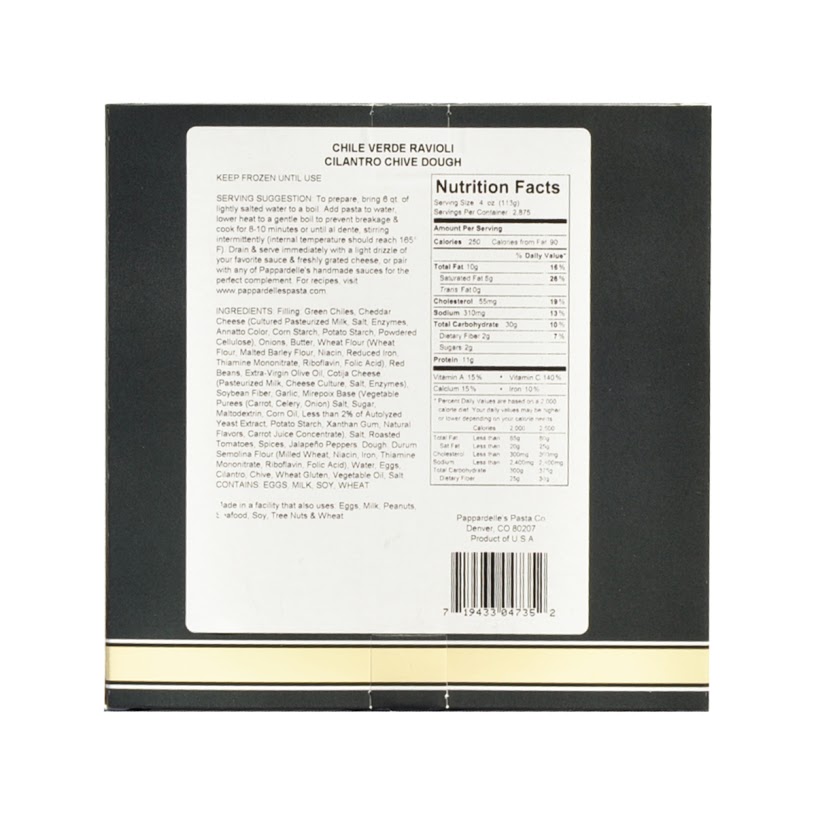This image displays a product label for Chili Verde Ravioli with Cilantro Chive Dough, affixed to what appears to be a predominantly blue box. The specific area framing the sticker features multiple horizontal lines: grayish, white, and blue, with varying thicknesses. The label, centrally placed, begins with "Chili Verde Ravioli" followed by "Cilantro Chive Dough."

On the left side of the label, there are detailed preparation and storage instructions. The label advises keeping the product frozen until use. Cooking instructions suggest bringing 6 quarts of lightly salted water to a boil, adding the pasta, then lowering the heat to a gentle boil to prevent breakage. The pasta should be cooked for 8-10 minutes or until al dente, stirred intermittently, ensuring an internal temperature of 165 degrees Fahrenheit before draining and serving immediately with a light drizzle of your favorite sauce and freshly grated cheese, or pairing it with any of Pappardelle's Handmade sauces. There's also a web address provided for recipes: www.pappardelleasta.com. Below these instructions, an ingredients list and an allergen notice indicate the product is made in a facility that processes eggs, milk, peanuts, seafood, soy, tree nuts, and wheat.

On the right side of the label, a rectangle with the heading "Nutritional Facts" contains nutritional information in black lettering. The label specifies a serving size of 4 ounces, serving per container 2.875, with 250 calories per serving, 90 of which are from fat. The total fat content appears to be 10 grams, approximately 18% of the daily value. Additionally, there is an address and a black QR code below the nutritional information block, although the text here and other nutritional details are difficult to read.